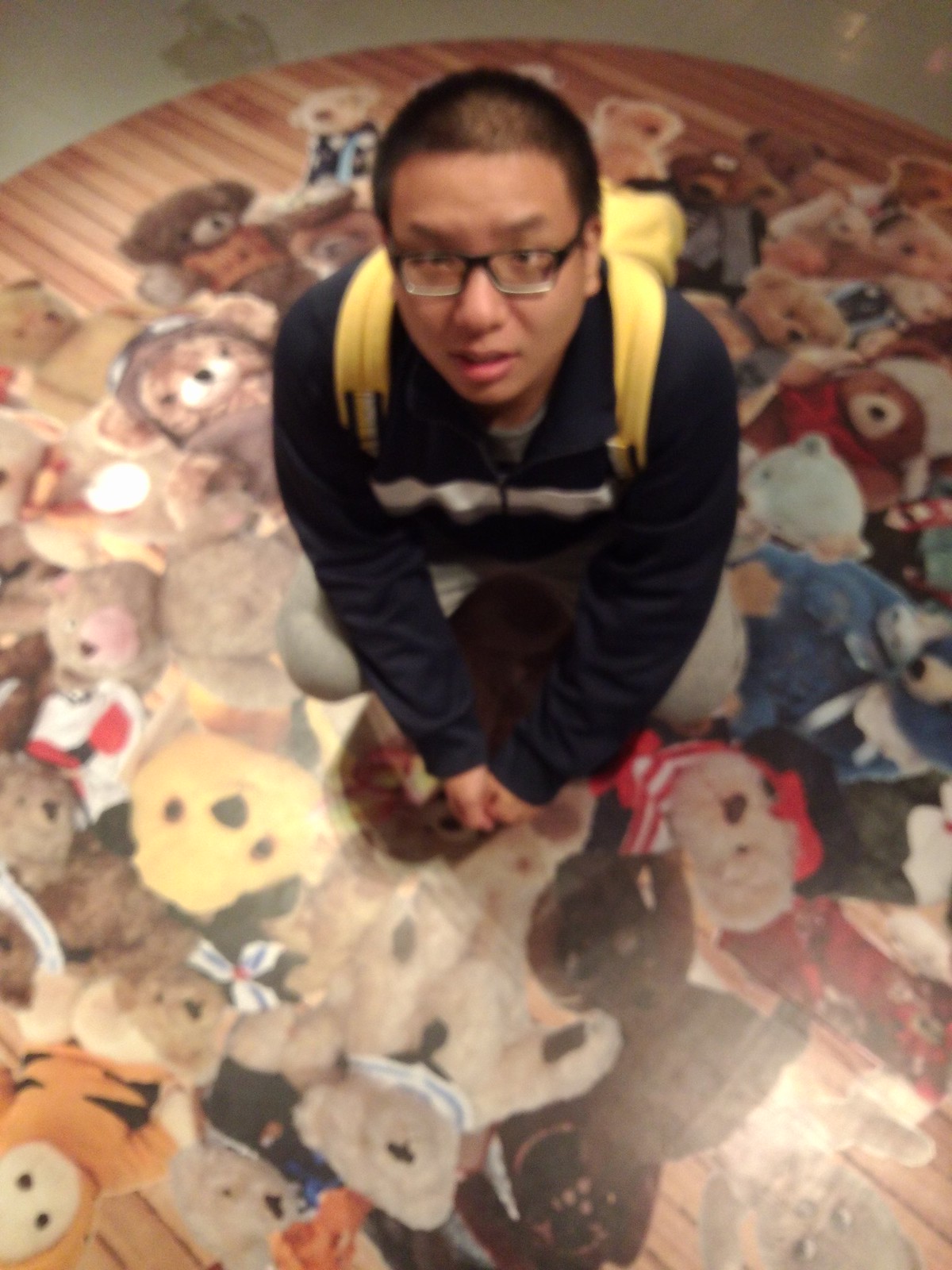The image captures a man of Asian descent, crouched down and looking up at the camera with a surprised expression on his face. He has very short, close-cut black hair and is wearing glasses. His outfit consists of a long-sleeve navy blue sweatshirt with a white stripe across the chest, paired with light brown or grayish pants. A bright yellow backpack is slung over his shoulders. He is situated on a round mat or piece of flooring adorned with an array of teddy bears in various shapes, sizes, and colors. The teddy bears are dressed in different outfits and feature a diverse palette, including brown, red, tiger-striped orange, tan, white, blue, and yellow. The background also shows a grey flooring area with a noticeable dark stain in the left-hand corner.